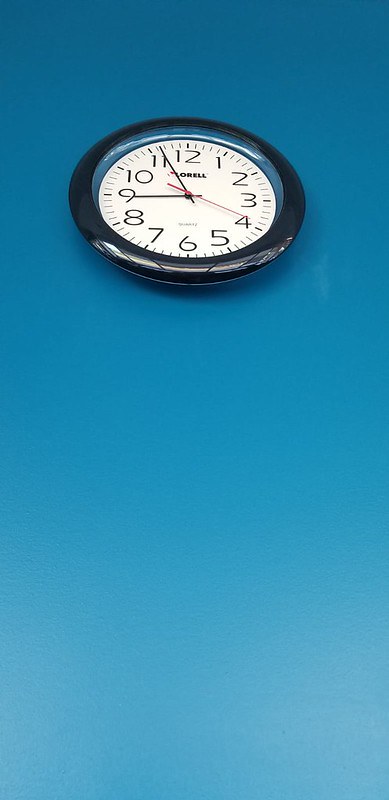"A vertical image captures a wall clock against a turquoise blue background. The clock, likely of the Dell brand, features a sleek, wide-rounded black frame and a classic white face. It displays standard black numerals and intermediate markings encircling the face. Narrow black minute and hour hands, complemented by a striking red second hand, indicate the time as 8:56. The perspective of the photograph gives the impression of looking up at the clock, offering a unique and immersive viewpoint."